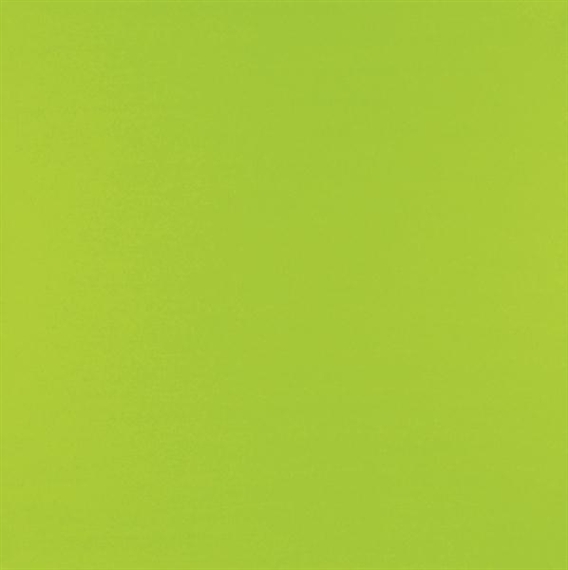The image depicts a plain, light green square featuring a uniform green color with no discernible variations or features. The shade is reminiscent of a pea green or a light, somewhat unappealing green akin to the color of vomit, though without any additional hues. The square is devoid of any patterns, lines, shadows, speckles, or other details. When observed closely, there may be a subtle hint of texture, potentially indicative of brush strokes, which suggests it could be a piece of modern art. However, this texture is not clearly defined and could also be a result of image resolution. The color appears slightly darker at the top and marginally lighter with faint yellow tones toward the bottom, but these differences are very subtle and almost imperceptible. Overall, the image remains a simple, solid green square.